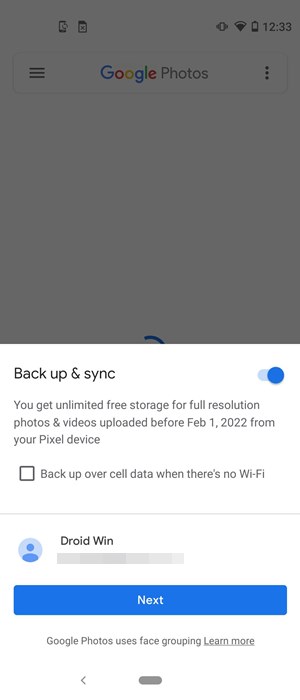The image is a screenshot taken from a smartphone, showcasing part of the Google Photos app interface. The top area of the screen features a translucent gray rectangle overlay, through which the background is faintly visible. Within this gray bar, the text "Google Photos" is prominently displayed. The time is shown as 12:33, and a battery icon on the right indicates a low battery level.

Beneath the gray bar, the main content area contrasts with either a white background at the top or bottom of the screen. Below the "Google Photos" label, a set of three vertical dots is present, indicating more options. The screen contains a message about backup and synchronization, stating "You get unlimited free storage for full-resolution photos and videos uploaded before February 1, 2022, from your Pixel device."

There is a toggle switch for the "Backup & sync" feature, which is currently enabled, indicated by a blue slider against a light white strip. Further down, there's an option labeled "Back up over cell data when there’s no Wi-Fi," associated with a checkbox. The text "Droid Win" is visible, likely indicating the device's name or an app feature. Finally, at the bottom right corner of the screen, a blue "Next" button is prominently displayed, offering a clear call to action.